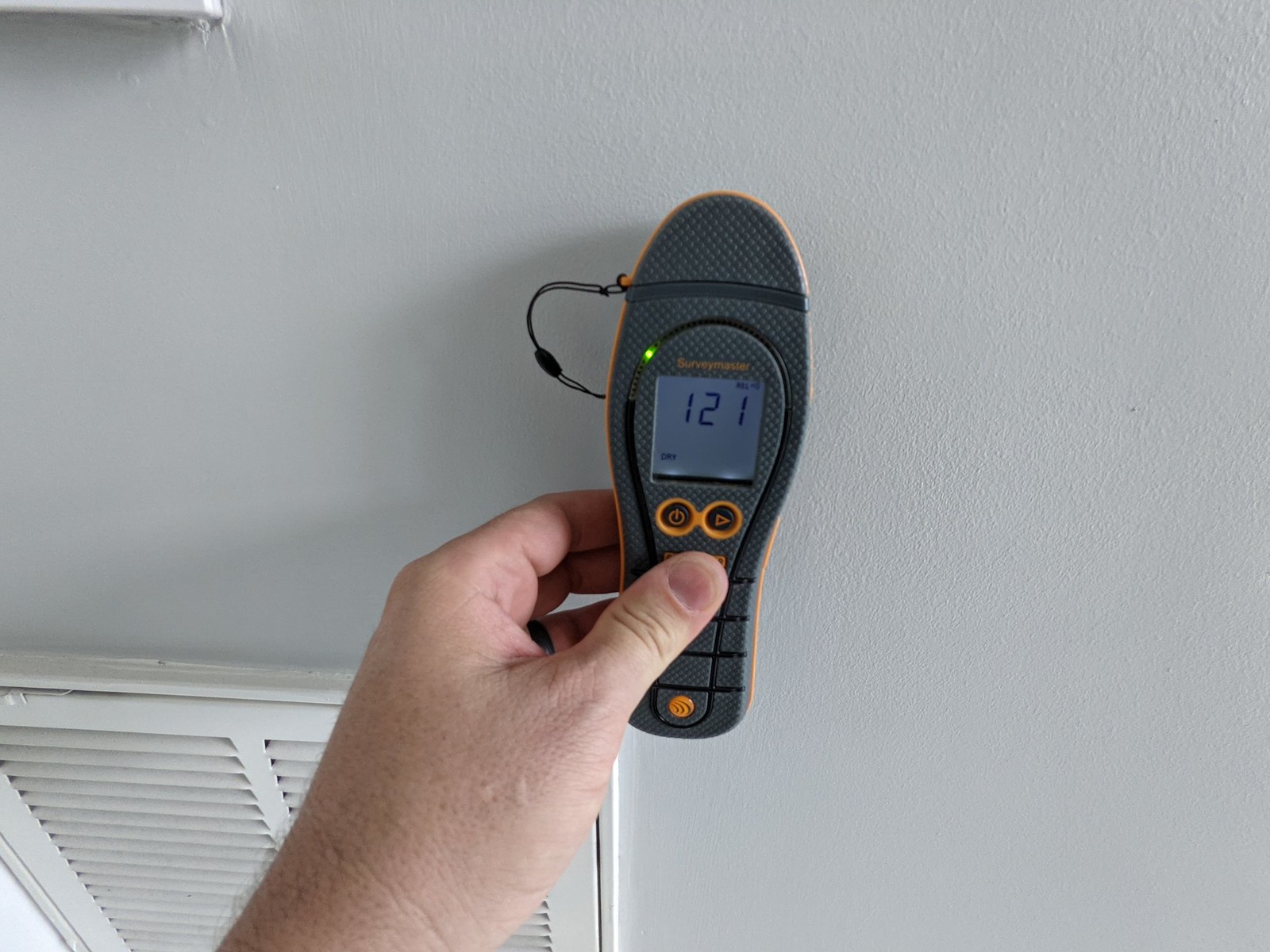In this detailed image, we observe a person using a handheld device with the brand name "Survey Master" engraved on it. The device is being pressed up against a white wall, prominently displaying a small square screen that shows the reading "121" and the word "Dry." There are two visible buttons beneath the screen: a power button and another button featuring a right-pointing triangle arrow.

In the bottom left corner of the image, part of an air vent panel is visible. A hand emerges from this side of the image, holding what appears to be the sole of a shoe. The "Survey Master" device itself is primarily gray with orange accents, including an orange outline and details around the buttons. At the base of the device, there's an additional orange symbol with three lines traversing through it, likely part of the brand's logo. In the upper left corner of the image, a small segment of a window sill is also visible, adding to the context of the indoor setting.